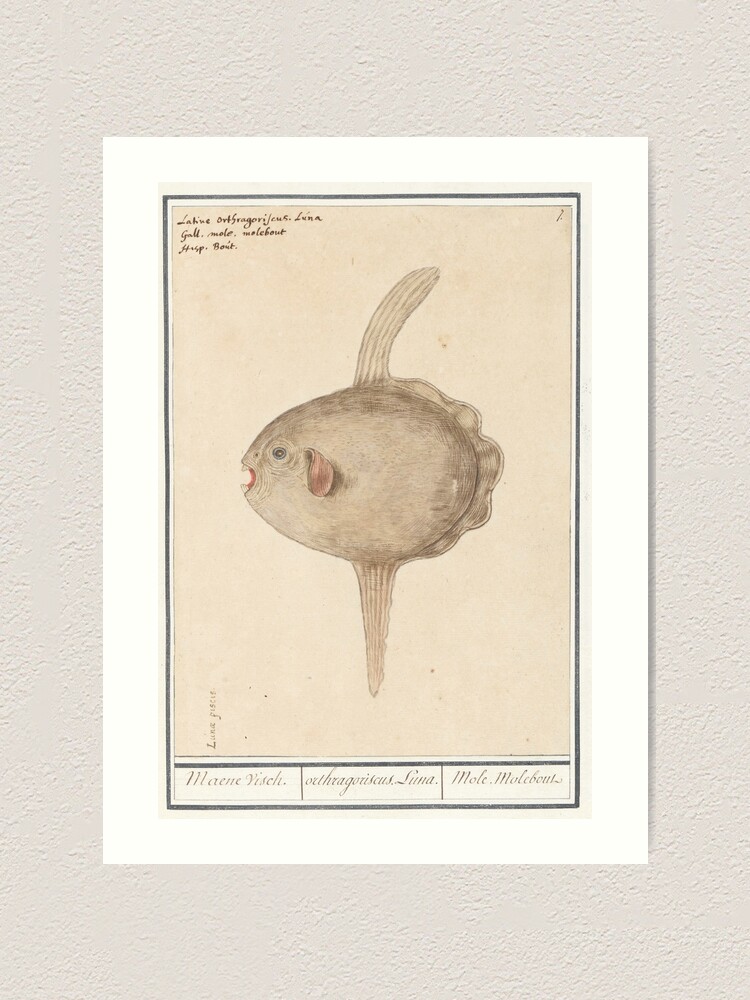The image depicts an old sketch or painting of a peculiar fish, framed and hung on a light greyish wall. The artwork, drawn on an off-white piece of paper that has aged to a yellowish hue, shows a fish with an egg-shaped body and a pair of unusual, elongated fins. The top fin, slightly thicker and curving to the right like a banana, contrasts with the straight, thin fin at the bottom. The fish’s bizarre features include a distinctive mouth. The sketch has a border around it, suggesting it’s mounted on the paper, and the entire piece is housed in a frame with a thick white border. Text appears in cursive in the top left corner and along the bottom, possibly indicating the species name or the artist’s signature, though it is difficult to read due to the photo's resolution and the faded ink.